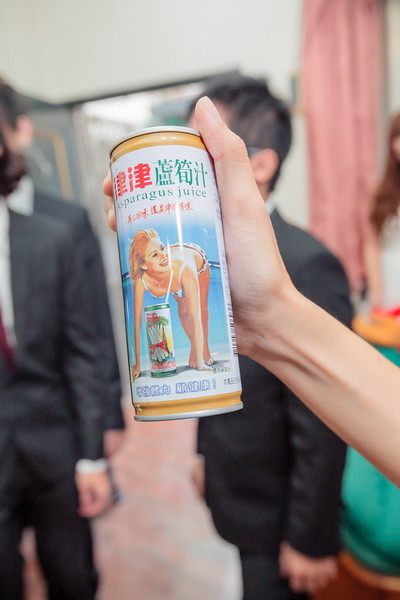The image depicts a can of asparagus juice, likely sourced from an Asian marketplace, as suggested by the presence of Asian characters on the label. The can features the words "Asparagus Juice" prominently displayed in English below the foreign script. Accompanying the text is a professionally hand-drawn illustration of a lady with blonde hair, and a smaller depiction of another can of asparagus juice. In the foreground, a person is holding the can towards the camera, enhancing its visibility. In the background, two individuals dressed in suits can be seen standing, adding a formal element to the scene.